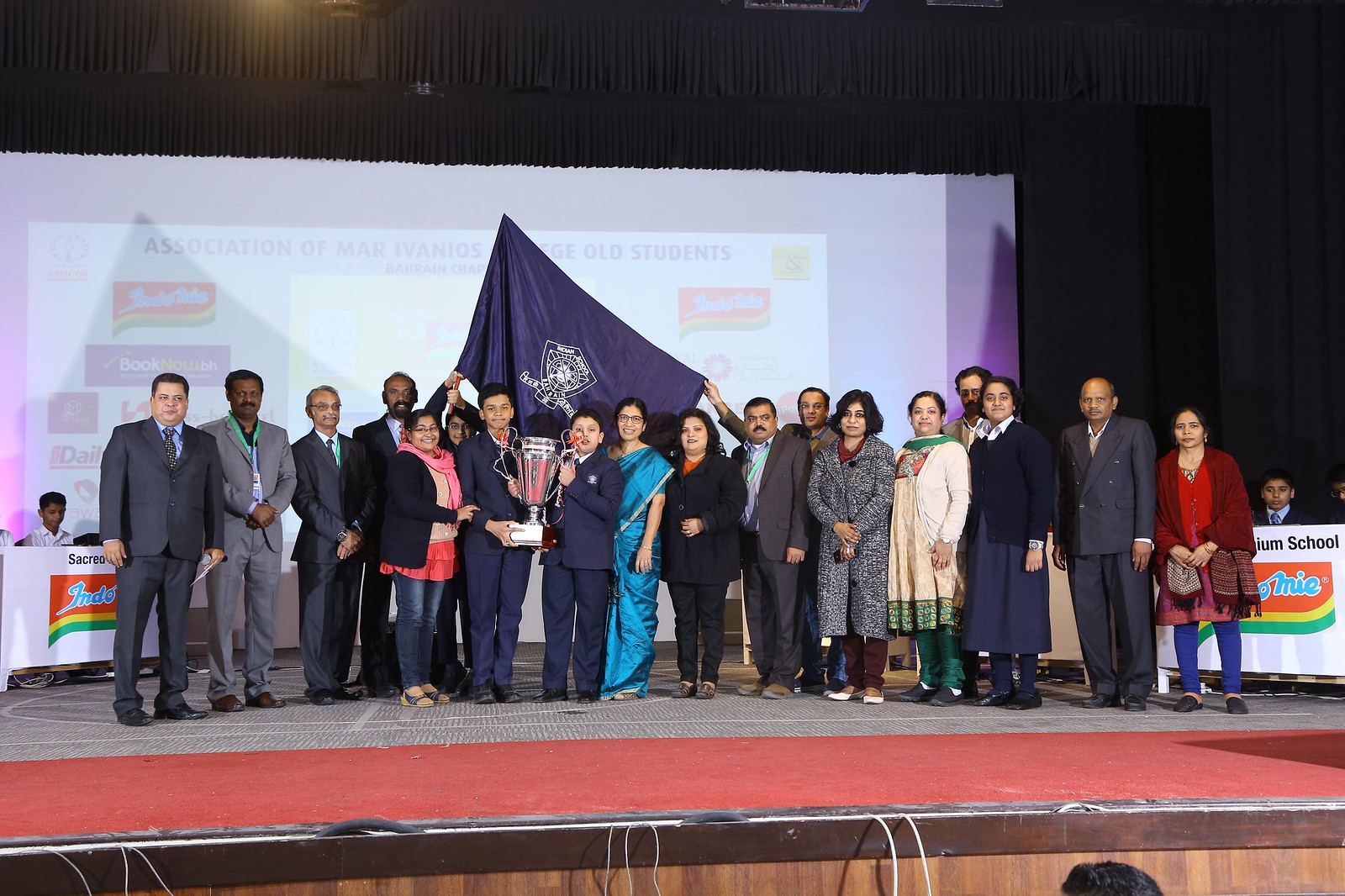This vivid full-color photograph captures an award ceremony taking place on a distinct stage in India, as denoted by the sign and traditional attire. The stage hosts an assortment of well-dressed men, women, and young boys, presumably part of a school event. Central to the scene are two boys holding up a large trophy, symbolizing their achievement. Behind the group, a blue flag with a golden emblem, though its details remain indistinct, adds a sense of ceremony. The stage itself is predominantly a metal gray structure with a front edge possibly adorned with red carpeting. Flanking the group are two white tables, featuring banners with black and multi-colored designs or logos that are partially obscured by the assembled people. The men and women on stage wear suits and dresses, emphasizing the formal and celebratory nature of the event.